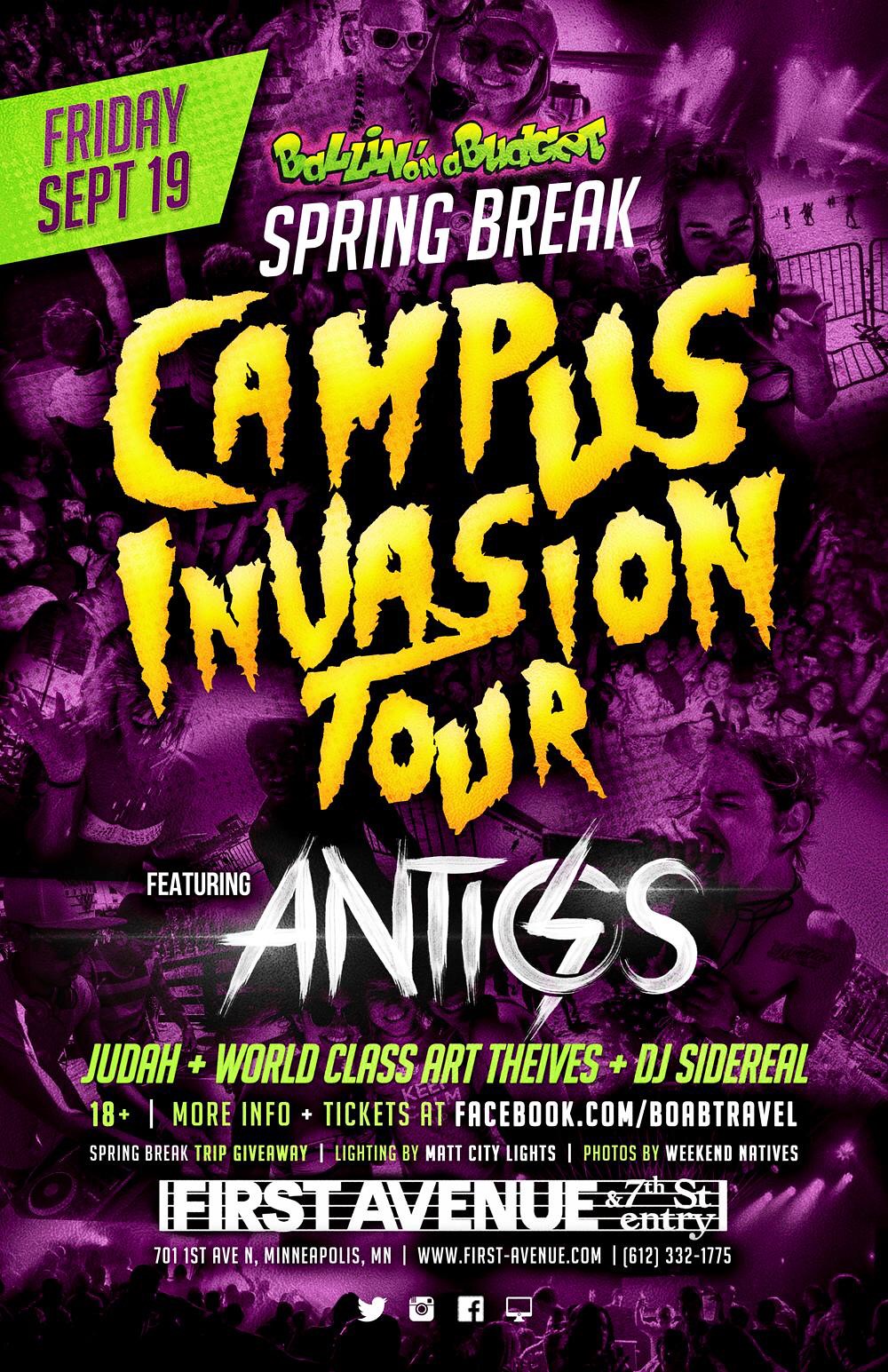This purple poster, designed with a collage-like background featuring numerous people creating a crowd, prominently announces an event. In the upper left corner, a green rectangular section with angled edges displays the date "Friday, September 19th" in purple font. Centrally positioned, the text "On a Budget, Spring Break" appears in green font, while the striking yellow "Campus Invasion Tour" title, styled in a Halloween-like font with a black outline, captures attention. Beneath this, "Featuring" is inscribed in a small white font, introducing the headliner "Antics," creatively written with a lightning bolt through the letter 'C'. Following are names of other performers in light green text: Judah, World Class Art Thieves, and DJ Sideral. The poster also specifies the event as 18+ and provides a call to action for more information and tickets at facebook.com/boabtravel. In the bottom section, it lists the venue details: First Avenue at 7th Street Entry, Minneapolis, Minnesota, and includes further address and contact information.